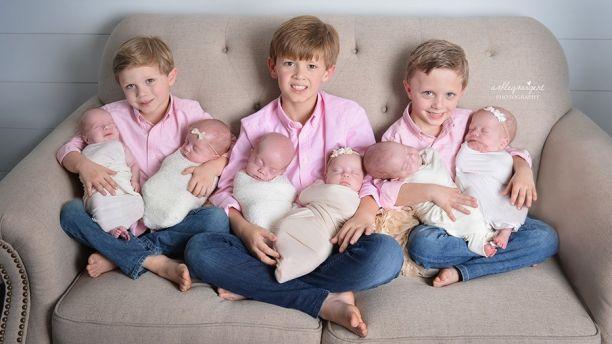The photograph captures a serene indoor setting where three young boys are seated cross-legged on a light brown couch, set against a gray wall. These boys, each with sandy blonde or light brown short hair, range in age from about 5 to 12 years old—the oldest in the middle appearing to be around nine, with the younger ones on either side. Dressed uniformly in slightly wrinkled, pink button-up collared shirts and blue jeans, their bare feet rest comfortably on the couch. Each of them cradles two tightly swaddled newborns, bringing the total to six babies—all of whom appear to be either siblings or close relatives. The newborns are bald with some adorned with little bows, with their eyes shut as though they are asleep. The boys’ smiles radiate warmth and joy, adding to the tender and familial atmosphere of the scene.